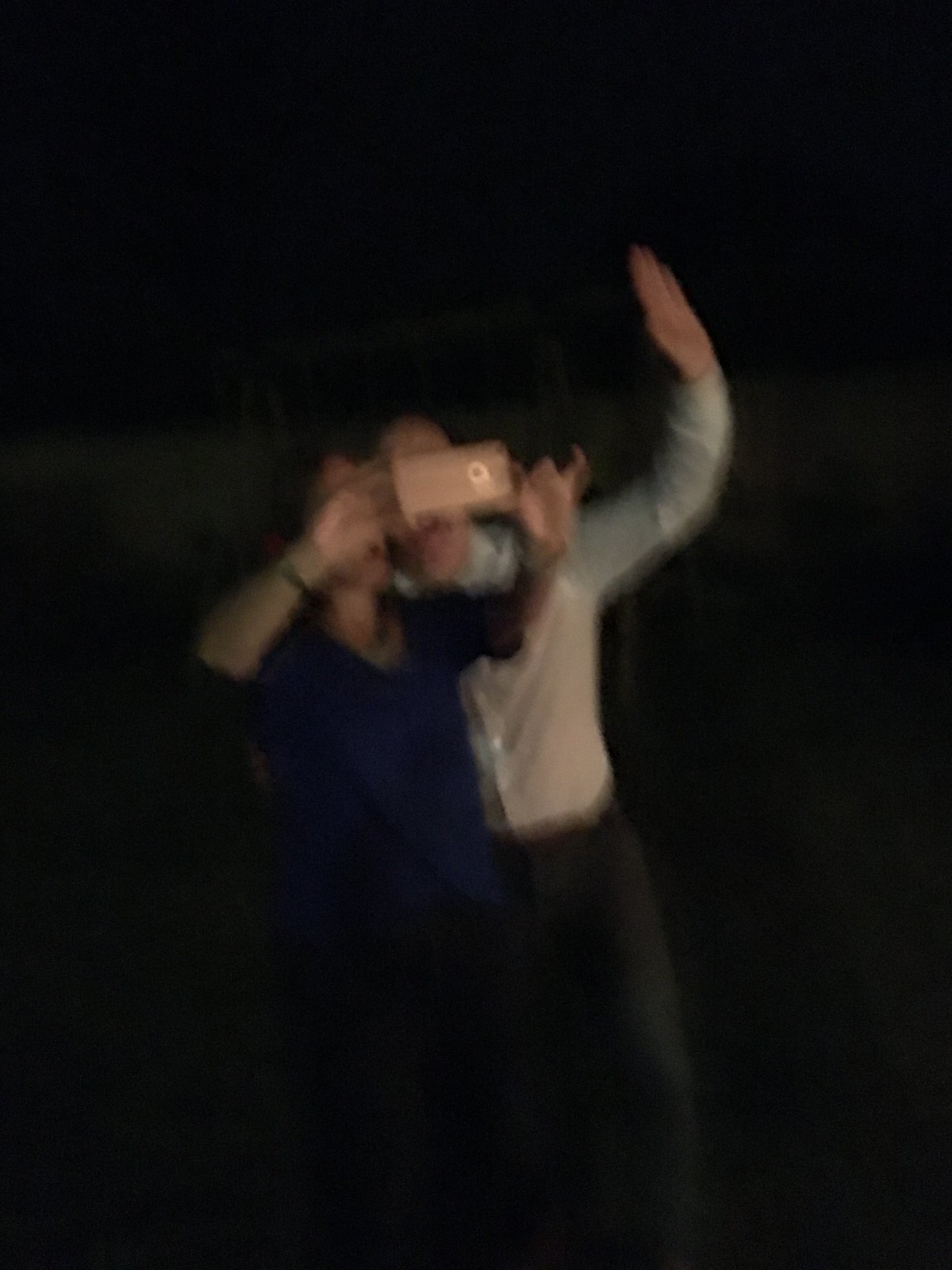The image is a blurry, grainy nighttime photo capturing two people outside, possibly in a backyard. The scene is dimly lit, with a faintly visible white fence and a grass-like surface underfoot. In the foreground, a woman with shoulder-length brown hair, wearing a deep blue blouse and black pants, is holding a pink iPhone horizontally as she takes a selfie. A man, standing to her right, is dressed in a light-colored long-sleeved shirt, a brown belt, and dark denim pants. He appears to be actively participating in the selfie, with his arm around the woman’s back. Their faces show open-mouthed smiles, indicating they are happy and engaged in the moment. In the dark background, an indistinct object resembling a swing set can be faintly seen, adding a touch of context to the outdoor setting.